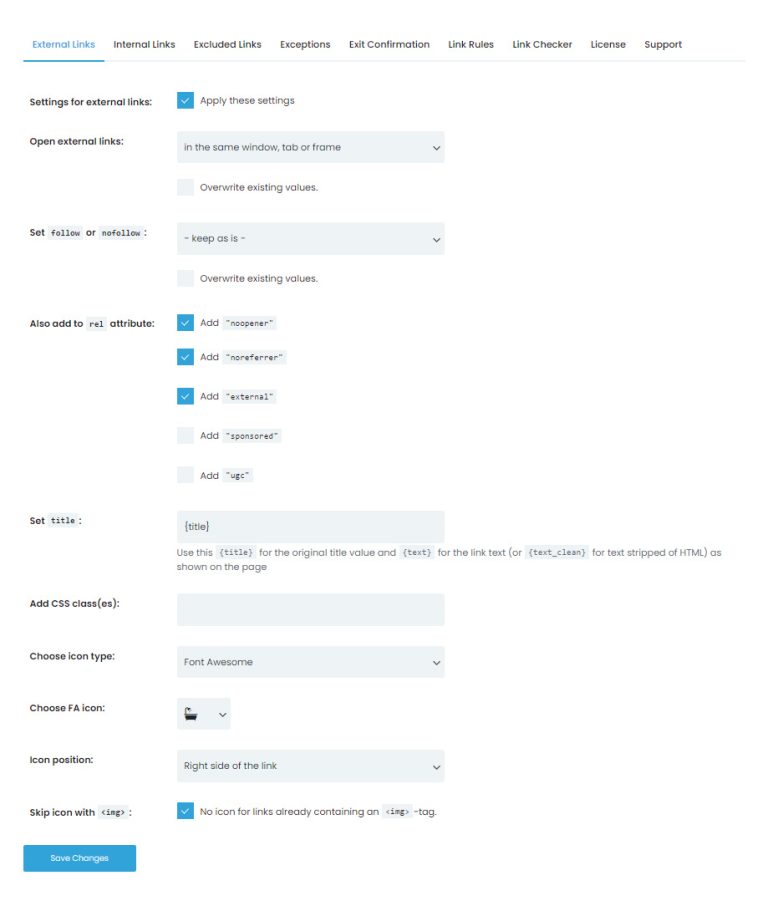The image depicts a computer screen displaying a webpage oriented towards link management settings. 

At the top of the page, a row of navigation tabs delineated by columns stands prominent. The tabs are labeled as follows: "External Links" (highlighted in blue), followed by "Internal Links," "Excluded Links," "Exceptions," "Exit Confirmation," "Link Rules," "Link Checker," "License," and "Support" (all displayed in black).

Beneath this row of tabs, a separator line divides the section containing the setting configurations. Immediately below this line is the header "Settings for External Links," alongside a blue checkbox labeled “Apply these settings.”

Following this header, the first major setting is titled "Open External Links," accompanied by a gray dropdown box that reads "In the same window/tab or frame." Adjacent to this is another gray box reading "Overwrite existing values."

The subsequent setting is "Set follow or no-follow," with a gray box labeled "Keep as is." Below this, another gray box is again labeled “Overwrite existing values.”

The next configuration section asks whether to add to the REL attribute, providing several blue and gray checkboxes: a blue checkbox for "Add 'noopener'," a blue checkbox for “Add 'noreferrer',” a blue checkbox for "Add 'external'," a gray checkbox for "Add 'sponsored'," and a gray checkbox for "Add 'UGC'."

Moving down, the following row addresses the title configuration with "Set Title (title)" in gray parentheses. It offers guidance stating, “Use this title for the original title value and text for the link text or text clean for text stripped of HTML as shown on the page.”

The next option pertains to CSS classes, marked as "Add CSS class or classes" with a subsequent gray field labeled "Choose icon." Below, the box reads “Font Awesome.”

Further down is "Choose FA Icon," presented with a gray box displaying a bathtub and shower symbol.

Continuing, the "Icon Position" setting is shown with a gray box displaying "Right side of the link."

The final row addresses skipping icons with "Skip icon with ING," with a blue checkbox corresponding to “No icon for links already containing ING tag.”

To finalize, a blue button at the bottom left of the page invites the user to "Save Changes."